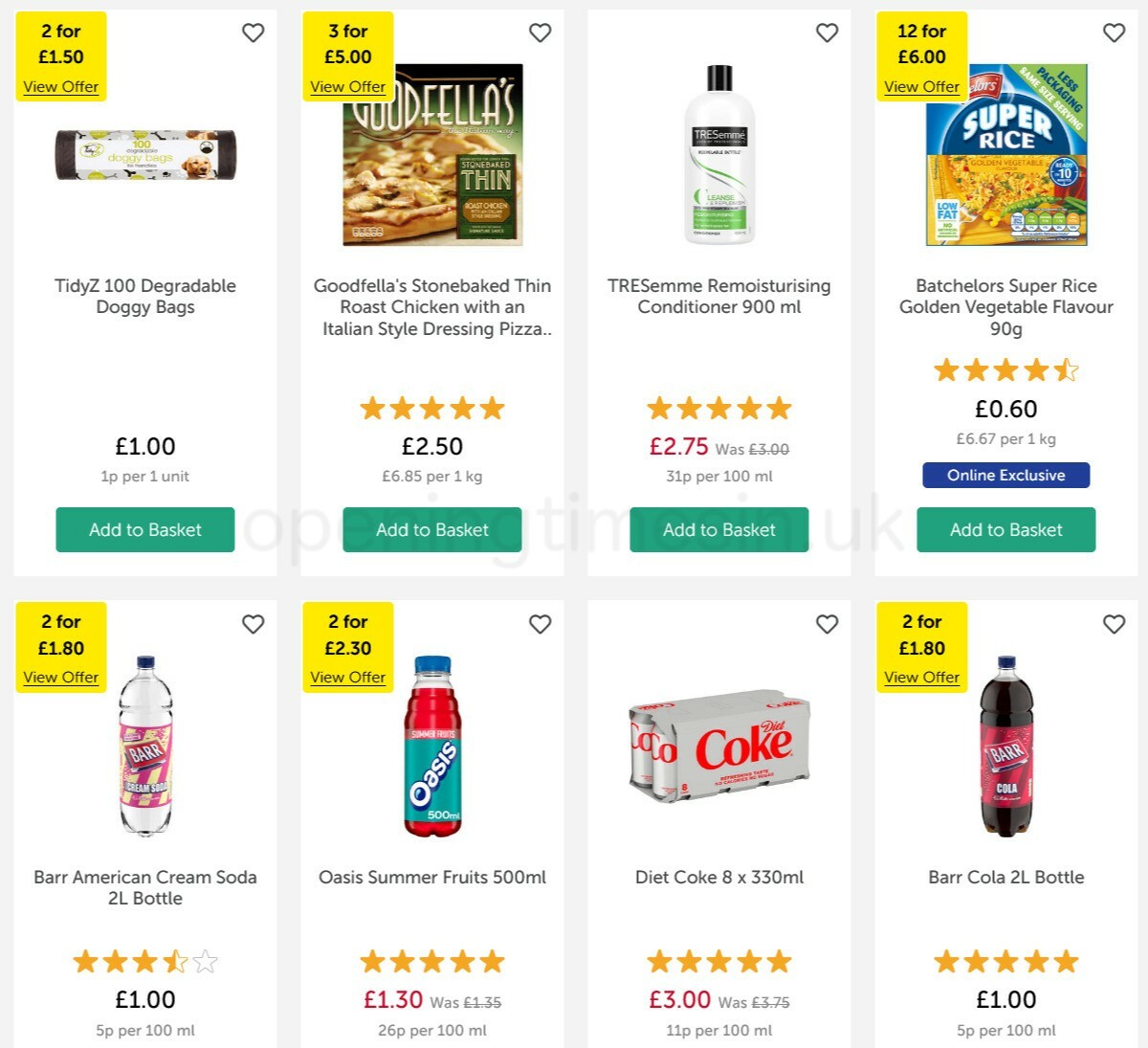An image of a computer screen from a grocery store displays eight rectangular product listings arranged in two rows. Each product listing includes details about the item such as prices, offers, and options to add items to the shopping basket. 

In the upper left corner, a yellow special offer box reads "2 for £1.50 view offer" for "Tidy Z 100 Degradable Doggy Bags," priced at £1 with an additional note of "1p per unit." There is an accompanying image of a circular container filled with dog bags and a green "add to basket" button.

Next to it is another yellow offer, "3 for £5 view offer," for the "Goodfellas Stone-baked Thin Roast Chicken with Italian-style Dressing Pizza." The pizza, priced at £2.50 (equivalent to £6.85 per 1kg), has an image of a frozen Goodfellas pizza, boasts a five-star rating, and includes a green "add to basket" button.

The third item is "Tresemme Conditioner 900ml," originally priced at £3, now reduced to £2.75 (31p per 100ml), and carries a five-star rating. It comes with a green "add to basket" button.

The final item on the top row offers "Bachelors Super Rice Golden Vegetable Flavor 90g" at 12 for £6. This item, priced individually at £0.60, includes an "online exclusive" label, a four-and-a-half-star rating, and a green "add to basket" button.

The second row begins with a "Bar American Cream Soda 2L" bottle, available at "2 for £1.80 view offer" in a yellow special box, priced at £1, and features a green "add to basket" button.

Next is "Oasis Summer Fruits 500ml," offered at "2 for £2.30 view offer" in yellow, priced at £1.30 (was £1.35), with a five-star rating and a green "add to basket" button.

The third item is an 8-pack of "Diet Coke 8x330ml" in silver and red packaging, priced at £3 in red text, also with a five-star rating and a green "add to basket" button.

Concluding the second row is a "Bar Cola 2L" bottle with a red label, offered at "2 for £1.80 view offer" and priced at £1, also featuring a five-star rating and a green "add to basket" button.